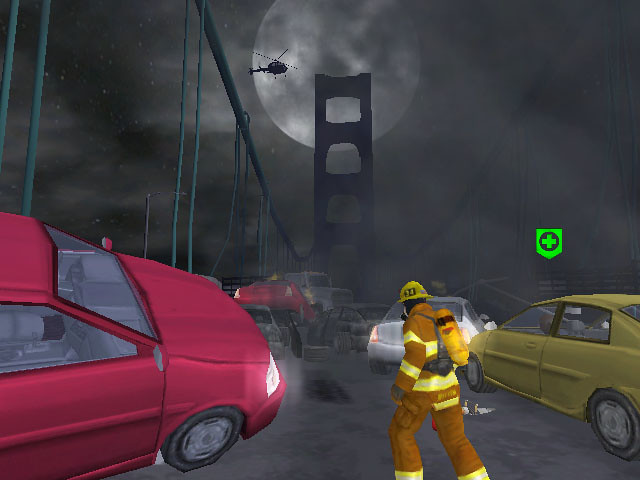In this nighttime scene enveloped in a smoky atmosphere, a fireman is standing on a bridge, responding to what appears to be a vehicular incident. Emerging from the left-hand corner of the photograph is the front and center portion of a reddish car, suggesting a possible crash or emergency. Dominating the sky is a large, luminous moon centered at the top of the image, casting an eerie glow over the scene. The pillar of the bridge rises prominently in the middle of the frame, framing the tense situation below. To further underscore the urgency, a helicopter is visible in the smoky sky, presumably part of the emergency response effort. The overall composition captures a moment of intense action and drama, framed by the infrastructure of the bridge and illuminated by the celestial body above.